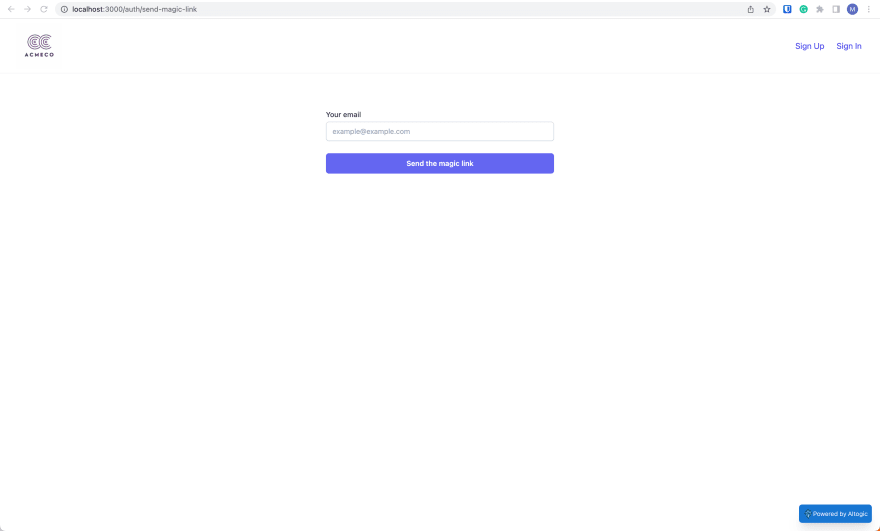This image is a screenshot of a web page, captured from a browser with the URL displayed in the address bar as "localhost:3000/auth/send-magic-link." The branding "Acme Co." is prominently displayed in the top left corner. On the opposite side, in the top right corner, there are links labeled "Sign up" and "Sign in." 

The central portion of the screen features a simple form with the label "Your email" set against a white background. Below this label is an input field placeholder that reads "example@example.com." Directly beneath the input field is a large purple button with the text "Send the magic link" in white, serving as a call-to-action.

The bottom right corner of the image bears the text "Powered by A-Logic," indicating the platform provider or developer. 

There are no other elements such as people, animals, plants, buildings, vehicles, or aircraft in the image. The focus is entirely on the user interface of the web page designed for email input and submission.